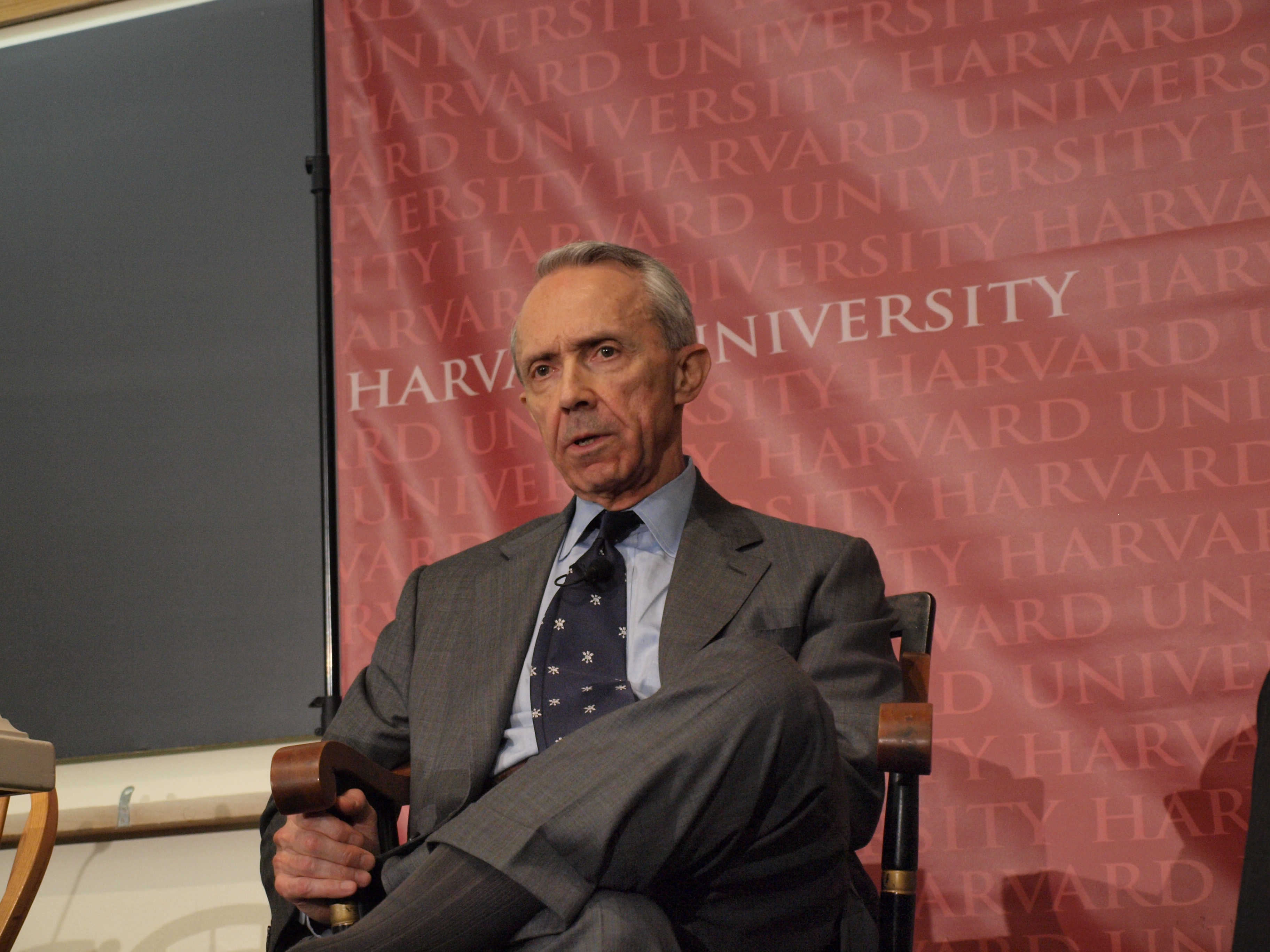In this image, a man wearing a gray suit, blue tie, and blue collared shirt is seated on a wooden chair, with gray socks visible. He has short, predominantly gray hair with some brown strands. The backdrop is a red banner or tarp that repeatedly says "Harvard University" in white or gray letters, in various shades of red and pink. Behind the man is a blackboard and another lighter-colored chair is partially visible next to him. The man is holding onto a part of the chair and looking downward. A shadow is cast in the bottom right corner of the image. Additionally, a microphone is attached to his tie.